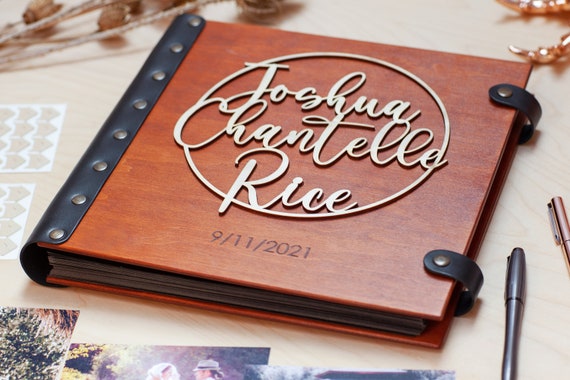This striking color photograph captures a beautifully crafted hardcover book at the center of the composition, potentially a journal or wedding album. The book features an elegant wood-like cover with two leather straps that snap from the back to the front, securing its contents. The spine is adorned with a black binding embellished with rivets, adding a touch of sophistication. Prominently displayed on the cover, a cutout reveals the name "Joshua Chantile Rice" and the date "9-11-2021," suggesting a personal or significant item. 

The book rests at an angle on a light tan, whitewashed wood table. Surrounding it are various items that enhance the narrative of the scene: two pens—one copper and one gunmetal—lie to the right of the book, while photographs peeking from the bottom left add a layer of sentimental value. Dried flowers are arranged at the top, complementing the rustic aesthetic. Scattered to the left center are stickers that appear to be punched out, and in the upper right corner, a long copper object partially enters the frame, adding a hint of intrigue to the composition.